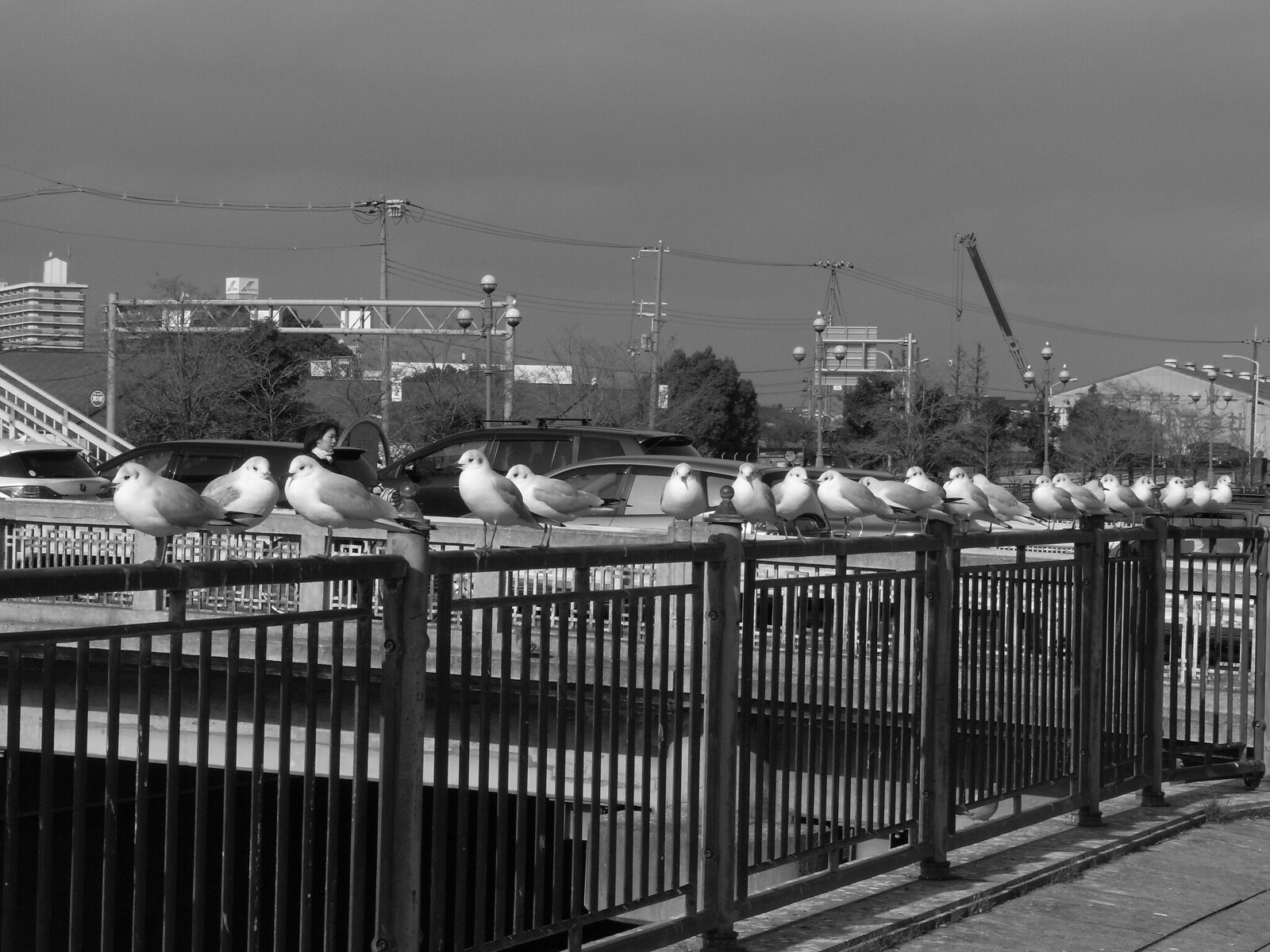A black and white photograph captures a diagonal wrought iron railing spanning from the bottom left to the lower right-hand side of the image. Perched atop the railing are approximately 20 seagulls and white-breasted pigeons, some facing the camera, others looking off into the distance. This scene is set against the backdrop of a bustling urban area. A cement bridge, visible in the mid-ground, crosses a riverway horizontally from left to right, with several cars and occasional pedestrians adding to the busy atmosphere. Further in the background, a complex array of train crossing lights and industrial train lights mark the area near a series of train tracks. Power lines, telephone poles, and streetlights crisscross through the scene, enhancing the dense cityscape ambiance. On a distant hill in the upper left corner, a multi-level high-rise building emerges from the horizon. Despite the intricate urban details, the sky remains a flat, murky gray, emphasizing the photo's monochromatic tone.